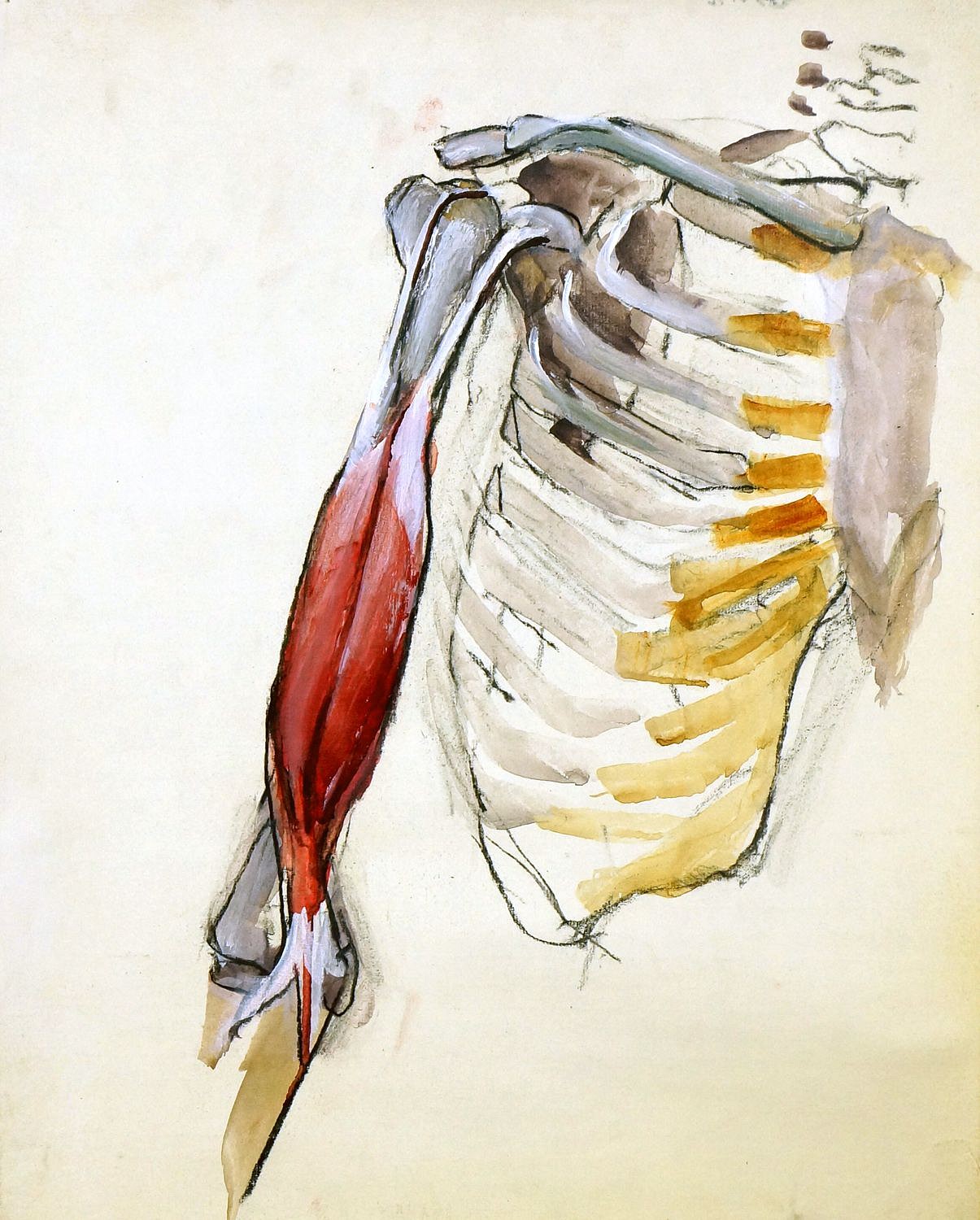This image features an abstract, smudgy painting of the right side of a human skeleton with elements of muscle and tendons. The medium of the artwork appears to be oil paint or a similar substance, creating a textured effect. Starting from the top, the neck area is painted with black and gray hues that suggest bones, possibly the neck bones, descending into a depiction of the ribcage. The ribcage is rendered in white and gray colors, with some sections highlighted in yellow on the right, hinting at the artist's focus on the bones' intricate structure. Below the collarbone, the structure extends to the humerus, depicted as a grayish-white bone. Unlike the complete skeletal representation elsewhere, the forearm is richly detailed with red-painted muscle strands, showcasing the connective white tendons leading to the wrist's gray bones. The background is a blend of brownish and white tones, adding depth and contrast to the central anatomical figures, giving the artwork a distinct and somewhat abstract appearance.